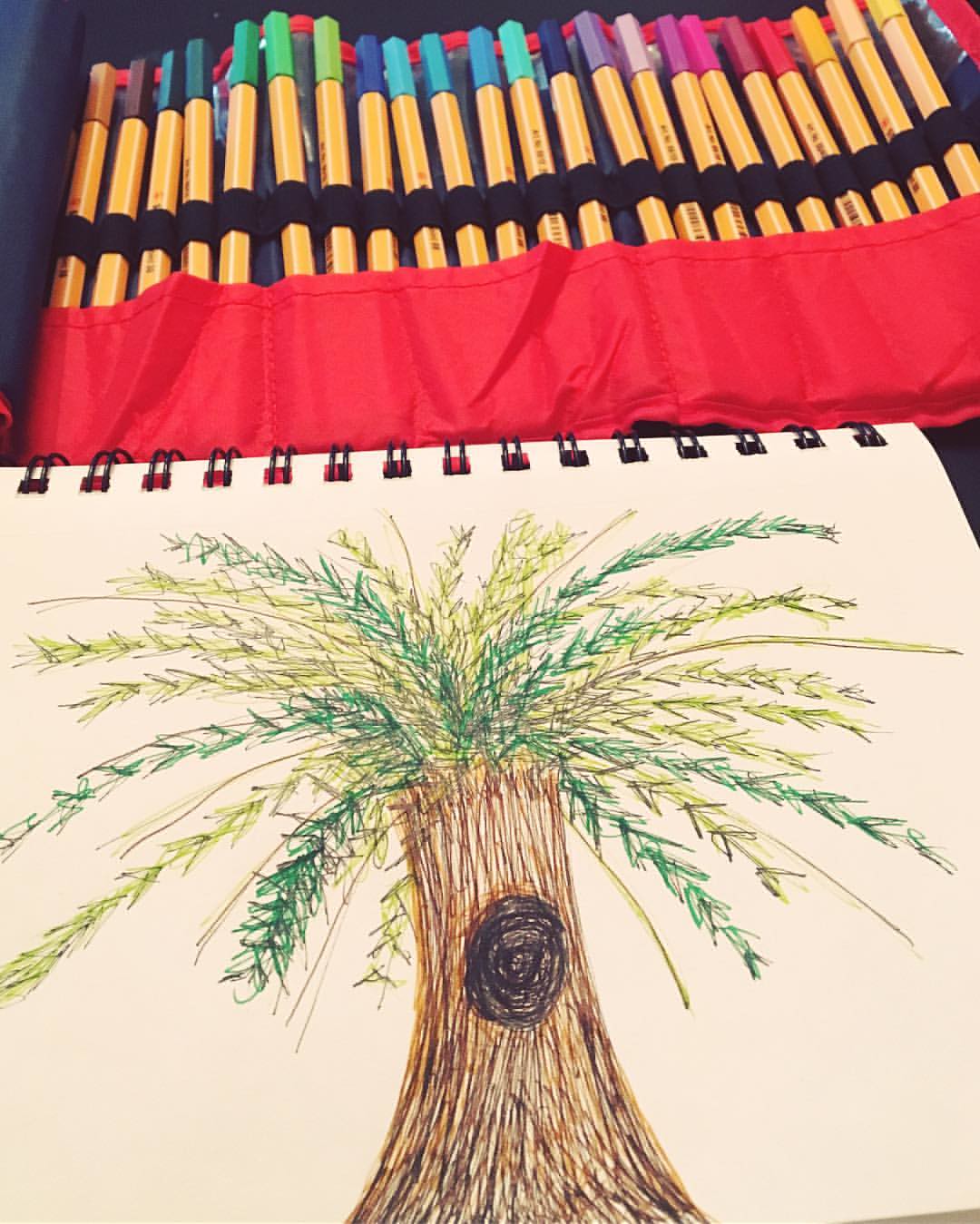This photograph captures a detailed drawing of a tree created using colored pencils. The illustrated tree features a prominent, robust main trunk, which includes a distinctive hollow at its center. From this trunk, numerous slender branches extend upward, each delicately drawn with a single line. These branches give way to a crown of leaves at the top, exhibiting a vibrant mix of dark and light green hues. Above the drawing pad, there is a red case meticulously organized with colored pencils, each pencil neatly placed in its designated slot.